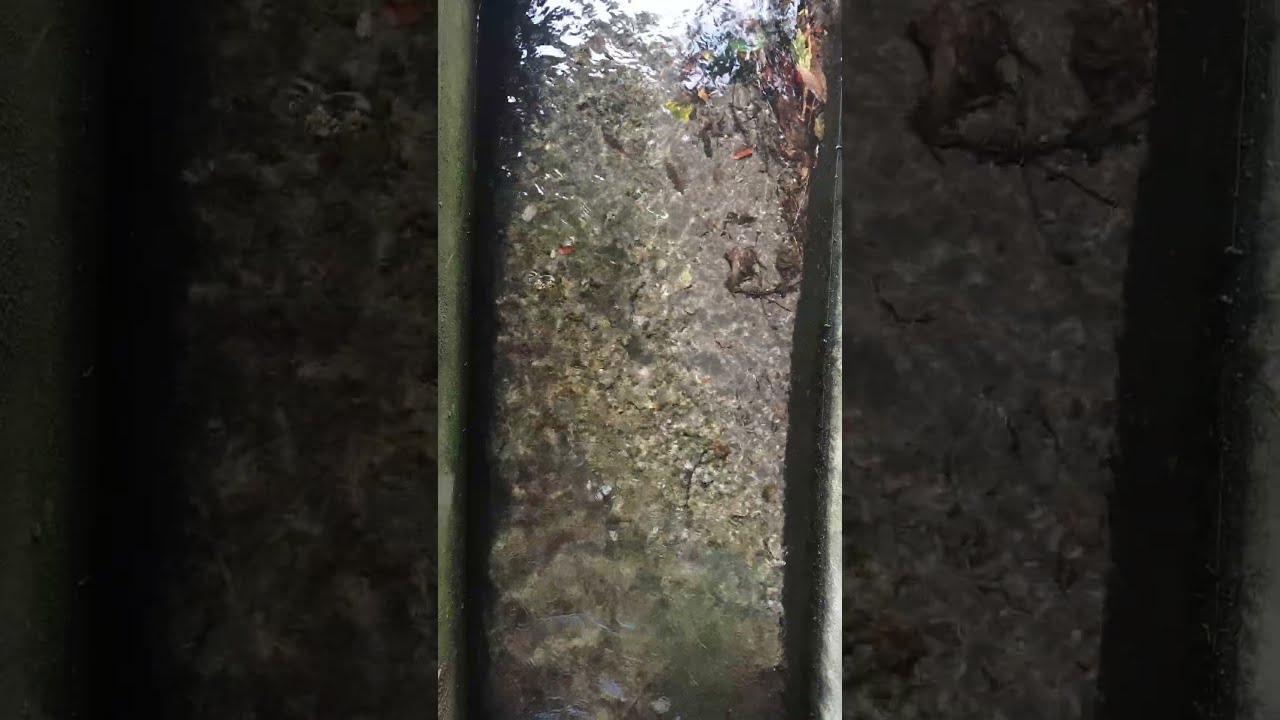The photo depicts a scene centered on a vertical, silver metallic drain pipe or storm pipe with dark shadows, resembling a gutter typically found in houses. The main image in portrait orientation is flanked by two zoomed-in, landscape-oriented insets showcasing detailed elements of the central pipe and its contents. The pipe appears cluttered with leaves, dirt, and debris, possibly submerged under water, contributing to a shadowy, darkened interior. The top of the pipe glimmers either from reflected light or the presence of refractive surface water, and leaves and fragmented debris are visible near the top of the setup. The overall photographic realism, coupled with nuanced lighting and shadowing, creates a detailed view of this seemingly clogged, nature-ensnared drainage system.